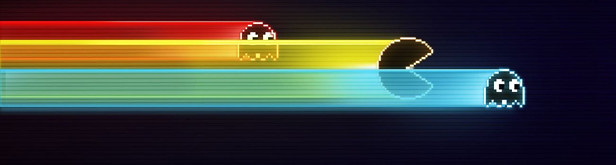A stylized graphic illustration reminiscent of a vintage video game, particularly Pac-Man, spans a rectangular space that is much wider than it is tall, with a solid black background. The image features three horizontal lines, each varying in length and color, streaking from left to right. The topmost line is a blend of red and orange colors, ending in a black ghost figure with round white eyes and black pupils, reminiscent of the ghosts from the Pac-Man game. Overlapping this, the middle line is yellow and showcases a Pac-Man figure - a circle with a wedge removed to depict its iconic mouth. The bottom-most line, the longest of the three, is blue and also features another black ghost figure with round white eyes and black pupils. Each element seems to move dynamically across the screen, capturing the fast-paced essence of the game.